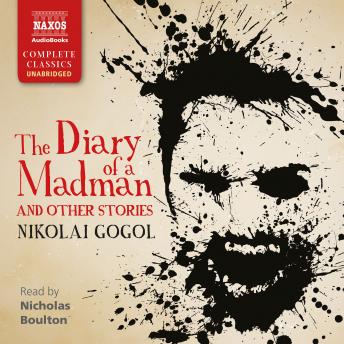This image features the square cover of an audiobook titled "The Diary of a Madman and Other Stories" by Nikolai Gogol. Dominating the right side of the cover is an intense illustration depicting a snarling madman with wild, black hair, a goatee, and frenzied black eyes against a beige background that darkens towards the edges. The textured appearance of the artwork resembles violent paintbrush strokes or ink splatters. The title, in vivid red handwritten text, appears on the center-left, while the author's name, Nikolai Gogol, is written immediately below in black text. In the lower right corner, it notes, “Read by Nicholas Boulton” in small gray text. The top left features a red badge with white text stating "Naxos Audiobooks," indicating the publisher, and below that, "Complete Classics Unabridged." The overall design suggests a compelling, auditory experience of Gogol's classic tales.